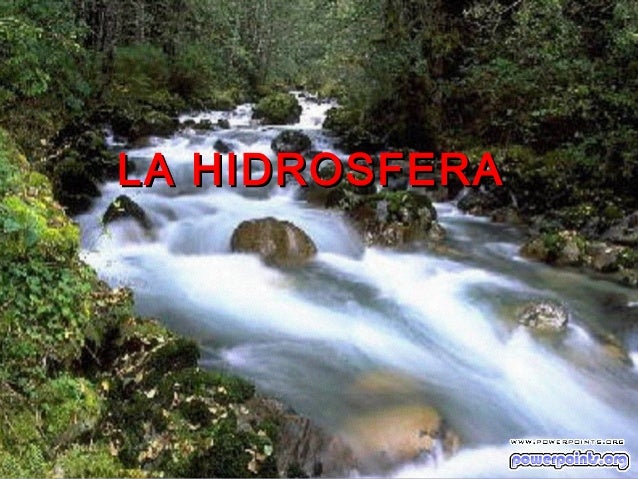The image is a somewhat blurry photograph depicting a dense, green forest with a fast-moving, foamy, white river winding through it. The river, strewn with large mossy boulders, originates from the top middle of the image and curves down towards the bottom right. The surrounding terrain is rocky and lush with dark green trees, evoking a rainforest-like atmosphere. Overlaid on the image, in all-capital red letters with black shadowing, is the Spanish word "La Hidrosfera." At the bottom right corner, the text "www.powerpoint.org" appears in black, with "PowerPoints.org" directly beneath it in blue.